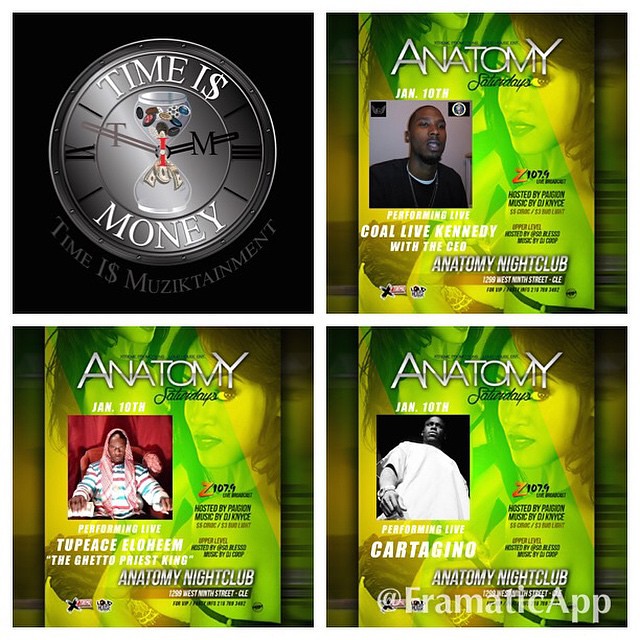The image is segmented into four equal squares, separated by white lines. In the upper left square, there is a black background featuring a silver metallic clock face with a shimmering effect. The clock displays Roman numerals and has white curved text that reads "Time is Money," with the 's' in "is" represented as a dollar sign. Additionally, an hourglass graphic transitions into dollar signs at the bottom of the clock.

The remaining three squares are essentially identical promotional posters, distinguished only by their different inset photographs. The background of these posters is green with lime yellow swirls and brown blobs at the corners. Across the top of the posters, white text reads "Anatomy Saturdays," and a heavily filtered image of an Asian woman with dark hair and lowering a strap on a negligee is visible in the upper right corner.

In the upper right poster, the inset photo features a young black male with a closely cropped hairstyle, a light mustache, and a dark shirt with a white collar. This square includes text about radio promotions and club details like dates and logos at the bottom. 

The lower left poster shows a young black man with long blonde hair and a striped sweater, seated in front of a red curtain. It mentions a performance by "Two Piece Elohim, the Ghetto Priest King" on January 10th.

The lower right poster displays a large, stocky African American male wearing a cut-off sleeve shirt, with a black background behind him, and mentions a performance by "Cartagena."

Each promotional poster includes similar details about the "Anatomy Nightclub," radio station Z107.4, and additional logos at the bottom.